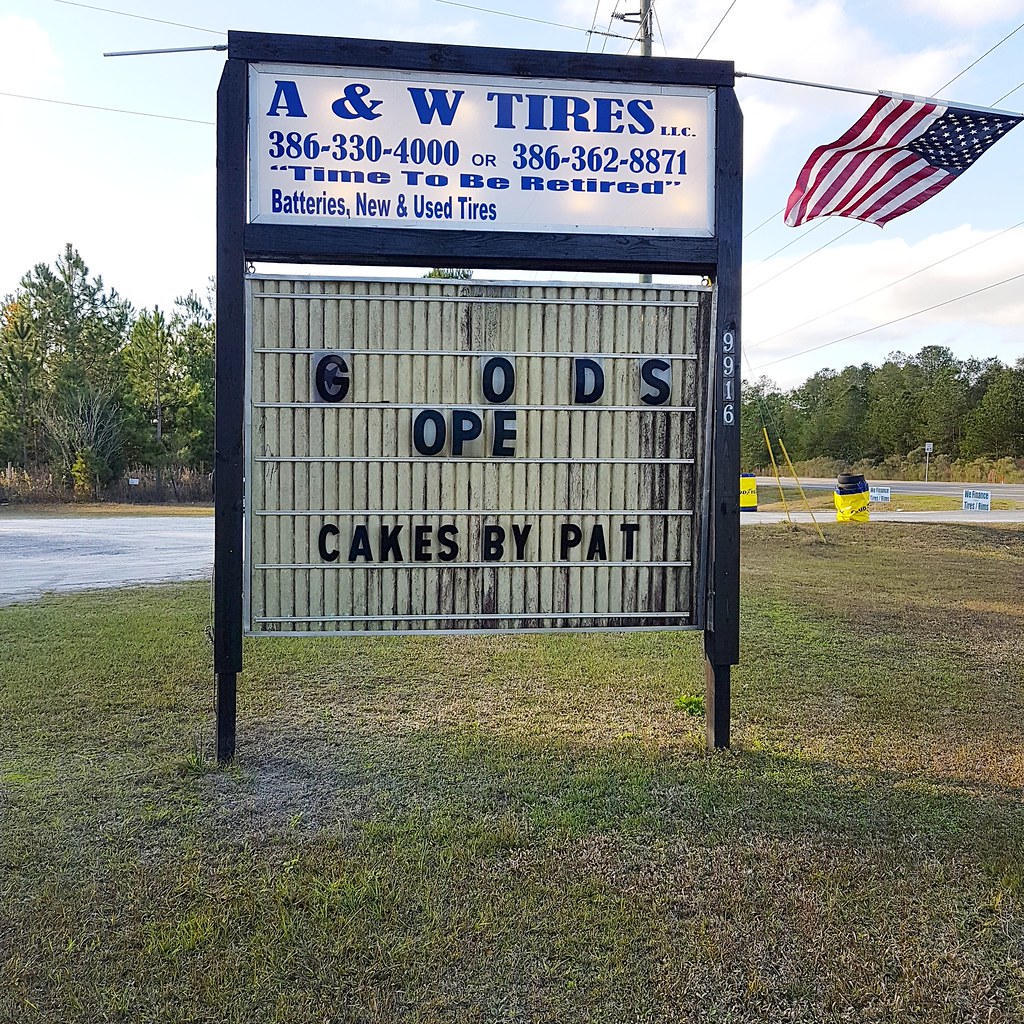This high-quality photograph captures a scene in a grassy area with predominantly light green and brown hues. Central to the image is a somewhat weathered sign. Portions of its letters have come off, leaving visible remnants: "G", "O", "D", and "S" on the top line, "O", "P", and "E" on the middle line, and below it, in black text, it reads "Cakes by Pat". 

Above this, there is a secondary sign featuring a white background with navy blue text that reads: "A&W Tires, 386-330-400 or 386-362-8871. Time to be Retired. Batteries, New and Used Tires". 

An American flag can be seen behind the sign, with trees and power lines stretching across the background, adding context to the location. The setting gives a rustic, small-town feel enhanced by the surrounding nature and elements of rural infrastructure.